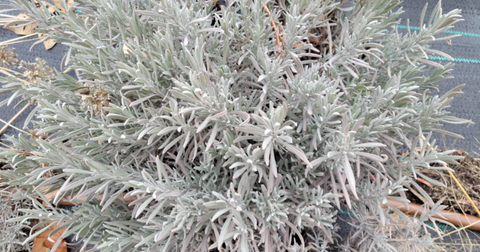This is a close-up, slightly blurry photograph of a pale, almost light gray plant with a dense, evergreen-like appearance. The plant features numerous branches extending in all directions, covered in tiny, sharp needle-like leaves that exhibit a very pale green coloration, frosted with white. These needles form a thick, lush, almost impenetrable foliage. The background reveals a dark paved asphalt surface with two thin teal-colored lines running horizontally across the upper part of the frame, predominantly visible in the top right corner, but also partially seen in the top left corner behind the plant. Below, in the bottom right, there's a small patch of brown dirt or sticks and a brown tube running from right to left across the bottom of the frame, mostly obscured by the plant. The overall scene suggests an outdoor setting, likely in a snowy environment, emphasizing the plant's striking, frosty appearance.